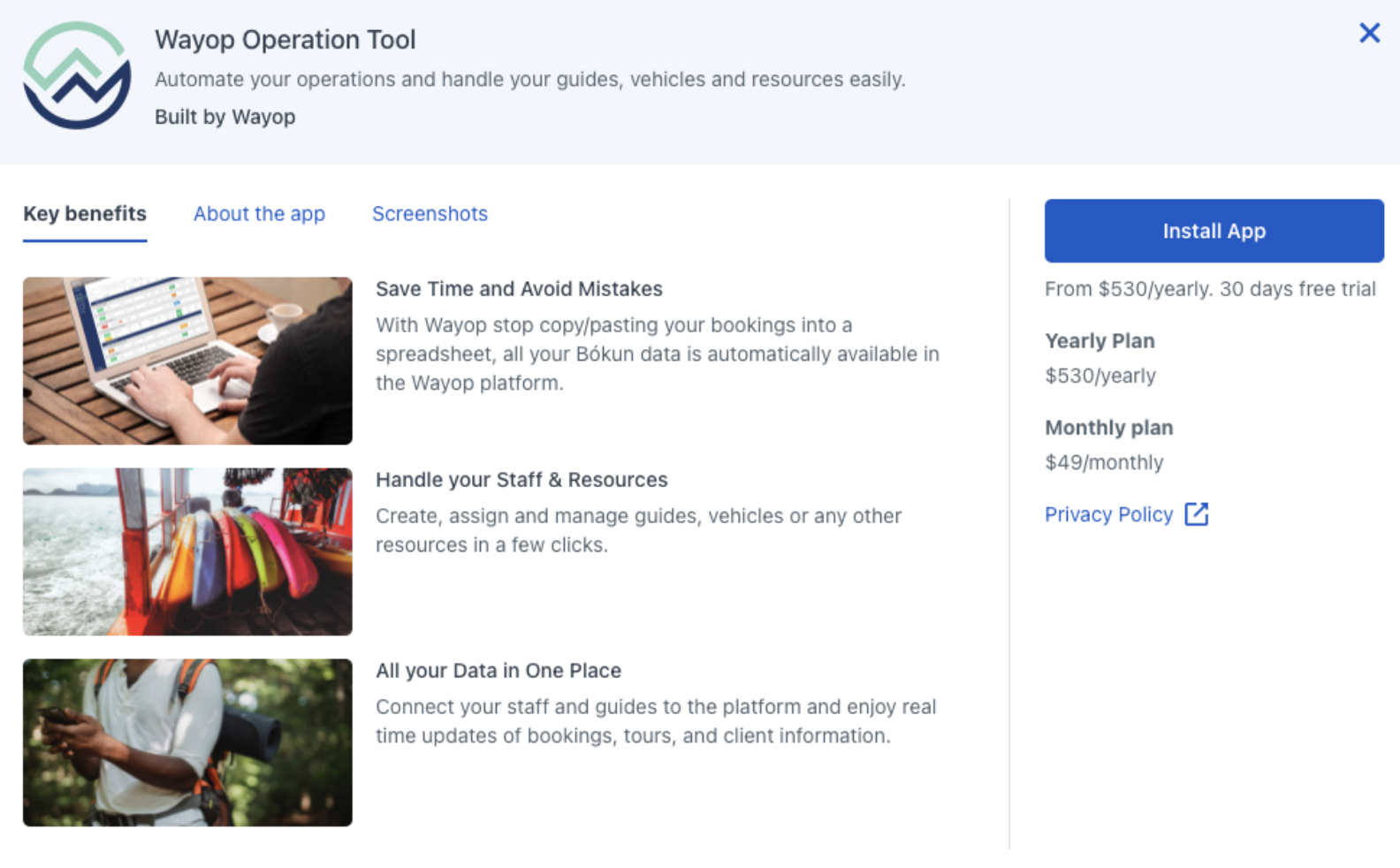In this image, we see a detailed display of the WayOp Operation Tool page. Dominating the interface is the title "WayOp Operation Tool" accompanied by the tagline, "Automate your operations and handle your guides, vehicles, and resources easily. Built by WayOp." In the upper right corner of the page, there is a small blue "X" button, allowing the user to close the tool.

There are three primary tabs visible, with the "Key Benefits" tab currently selected. This section features a breakdown of the tool's advantages:

1. **Save Time and Avoid Mistakes**: An informative description explains how users can stop copy-pasting bookings into spreadsheets, as all BOCUN data is automatically integrated into the WayOp platform, reducing errors and saving time.

2. **Handle Your Staff and Resources**: Users can effortlessly create, assign, and manage guides, vehicles, and other resources with just a few clicks, enhancing operational efficiency.

3. **All Your Data in One Place**: By connecting staff and guides to the platform, users can enjoy real-time updates on bookings, tours, and client information, streamlining communication and coordination.

On the right side of the page, a prominent blue button labeled "Install App" stands out, clearly indicating the next step for interested users. The cost of the app is outlined as $530 yearly, with a 30-day free trial available. Alternatively, there is a monthly plan priced at $49 per month. Additional clickable elements include a "Privacy Policy" button and a general interactive button.

Lastly, the interface includes tabs for "About the App" and "Screenshots," suggesting where users can find further information and visual previews of the app's features and interface.

Overall, this detailed breakdown of the WayOp Operation Tool's main page highlights its comprehensive functionality and user-centric design aimed at simplifying and automating operational tasks.